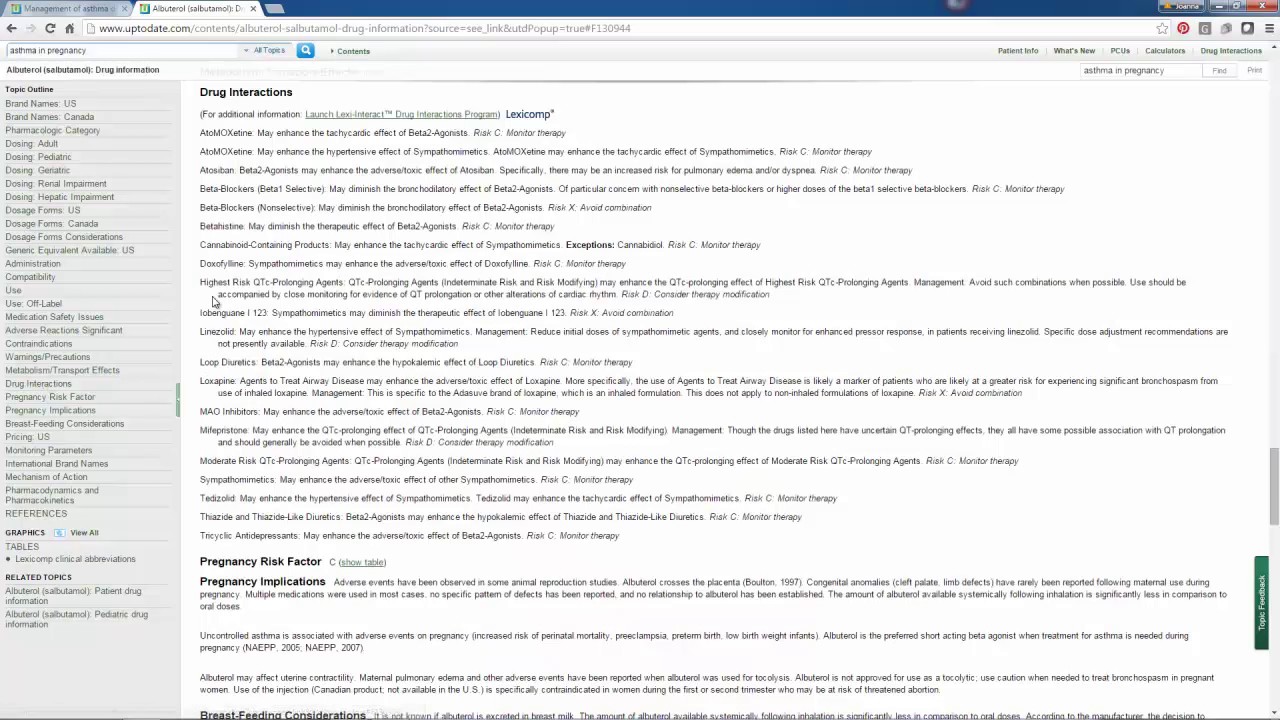Here is a refined, detailed caption for the image description provided:

---

This screenshot appears to have been taken from either a desktop computer or a laptop, showcasing a web browser window with two open tabs situated on the top left side. The webpage displayed has a predominant white background with a substantial amount of text content, some of which is formatted in bold. On the left-hand side, there is a vertically-oriented navigation menu, listing various chapters and links.

In the central section of the screen, extensive information is presented, featuring both bold and regular text styles against the white backdrop. The overall color scheme of the webpage is primarily black text on white, giving it a monochromatic appearance.

At the upper-right corner of the browser window, standard control icons for minimizing, maximizing, and closing the window are visible. The close button stands out as a rectangular shape with a red background and a white "X".

Additionally, several plugins and add-ons can be seen as small icons situated along the right side of the browser's address bar. There is a noticeable dark blue border running across the top of the webpage.

Underneath the two open tabs, a URL link is displayed in a combination of black and light gray text.

---